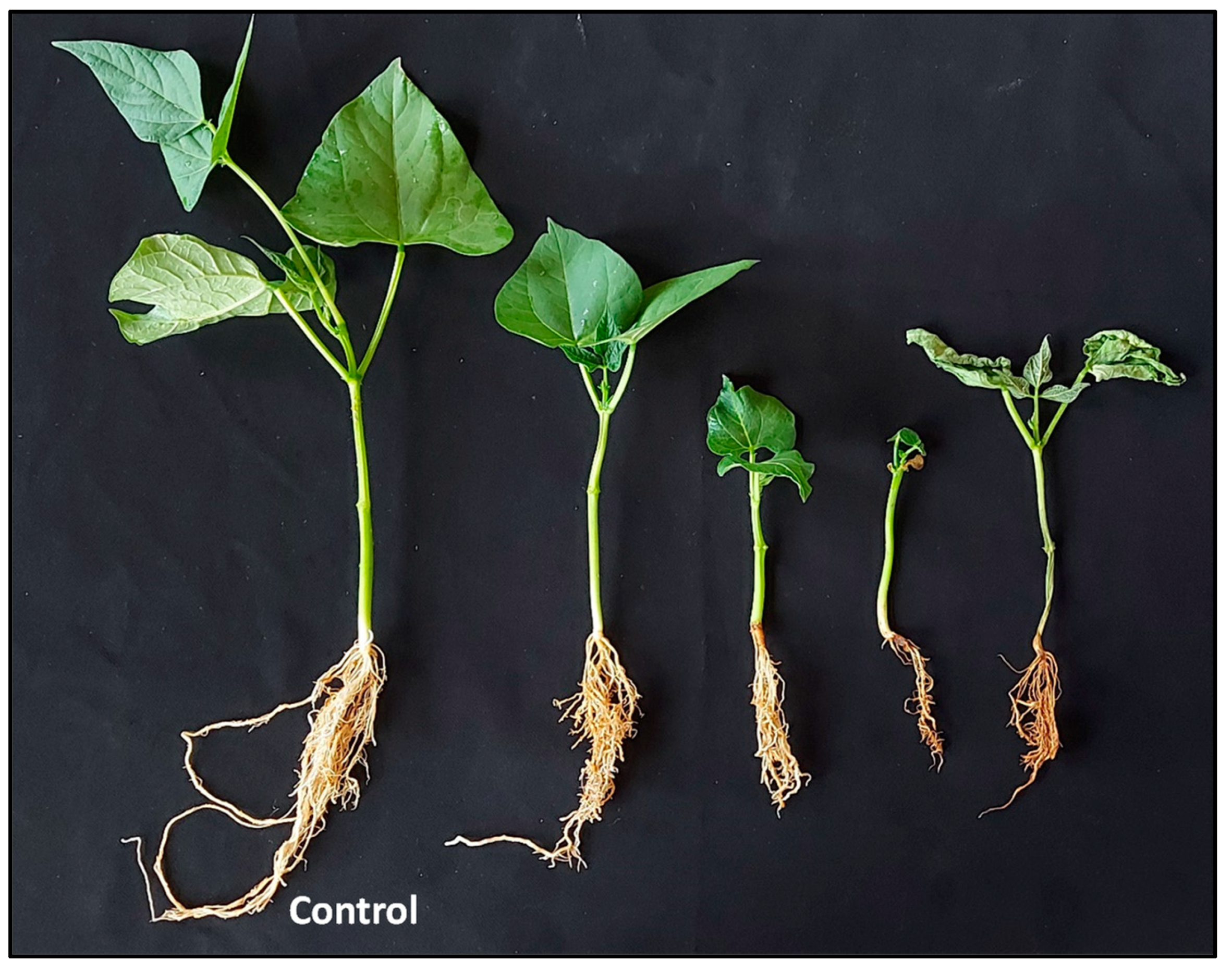The image depicts a horticultural experiment against a pure black backdrop, possibly a fabric or paper with visible creases. Center stage are five plants, likely of the same species, displayed in various stages of growth from left to right. These plants have been uprooted, showcasing their delicate white root structures beneath their stems. The far left, labeled "CONTROL" in white lettering, is the tallest, most well-developed plant with three or four green, pointed leaves. Each subsequent plant to the right is progressively smaller, with the second plant slightly shorter but still bearing three leaves. The remaining three plants demonstrate even less growth, their leaves smaller or nearly absent, and their roots less established. This orderly arrangement seems designed to illustrate the developmental variations under different conditions, underscoring the differences in size and health among the seedlings.